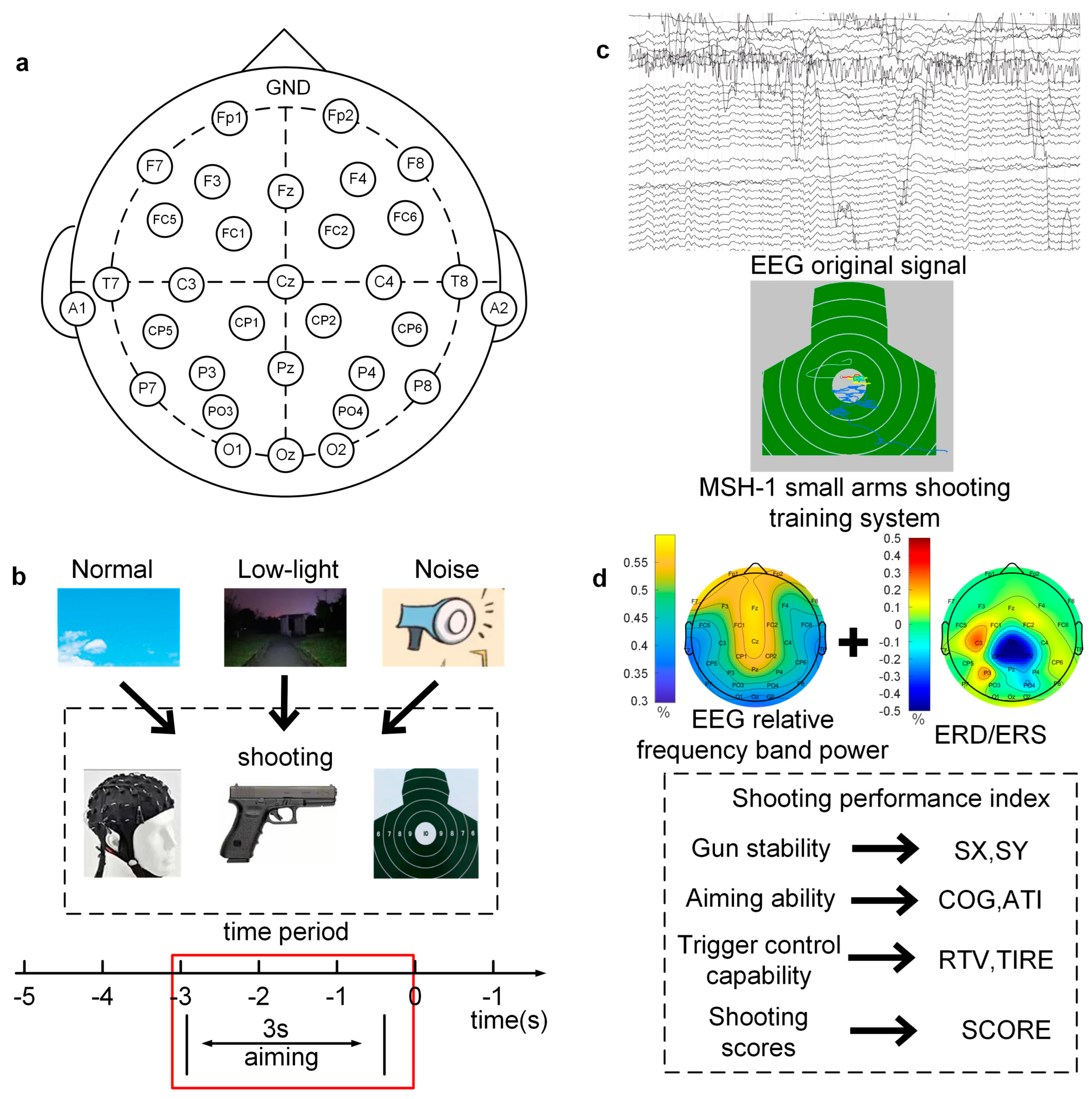The image presents a series of detailed charts and graphs related to small arms shooting training. The left side of the image, labeled A, shows a chart for GND with a circular layout. Adjacent to it, chart B illustrates different conditions: "normal" with a bright blue sky and white clouds, "low light" with a dark sky, and "noise" represented by a megaphone. Each condition points to various elements associated with shooting scenarios: "normal" points to a sculpture wearing a helmet, "low light" points to a gun labeled "shooting," and "noise" targets a man's heart depicted as a target. A time period of three seconds for aiming is indicated, with a red box marking between -3 and 0 seconds.

On the right side, section C is labeled "EEG original signal," featuring the MSH-1 Small Arms Shooting Training System and an EEG graphic. Section D is labeled "EEG relative frequency band power," showing ERD, ERS, and a shooting performance index. Together, these elements form a comprehensive graphic from an educational resource designed to assist with training and improving shooting accuracy and performance, incorporating visual aides and data on shooting conditions and physiological responses.